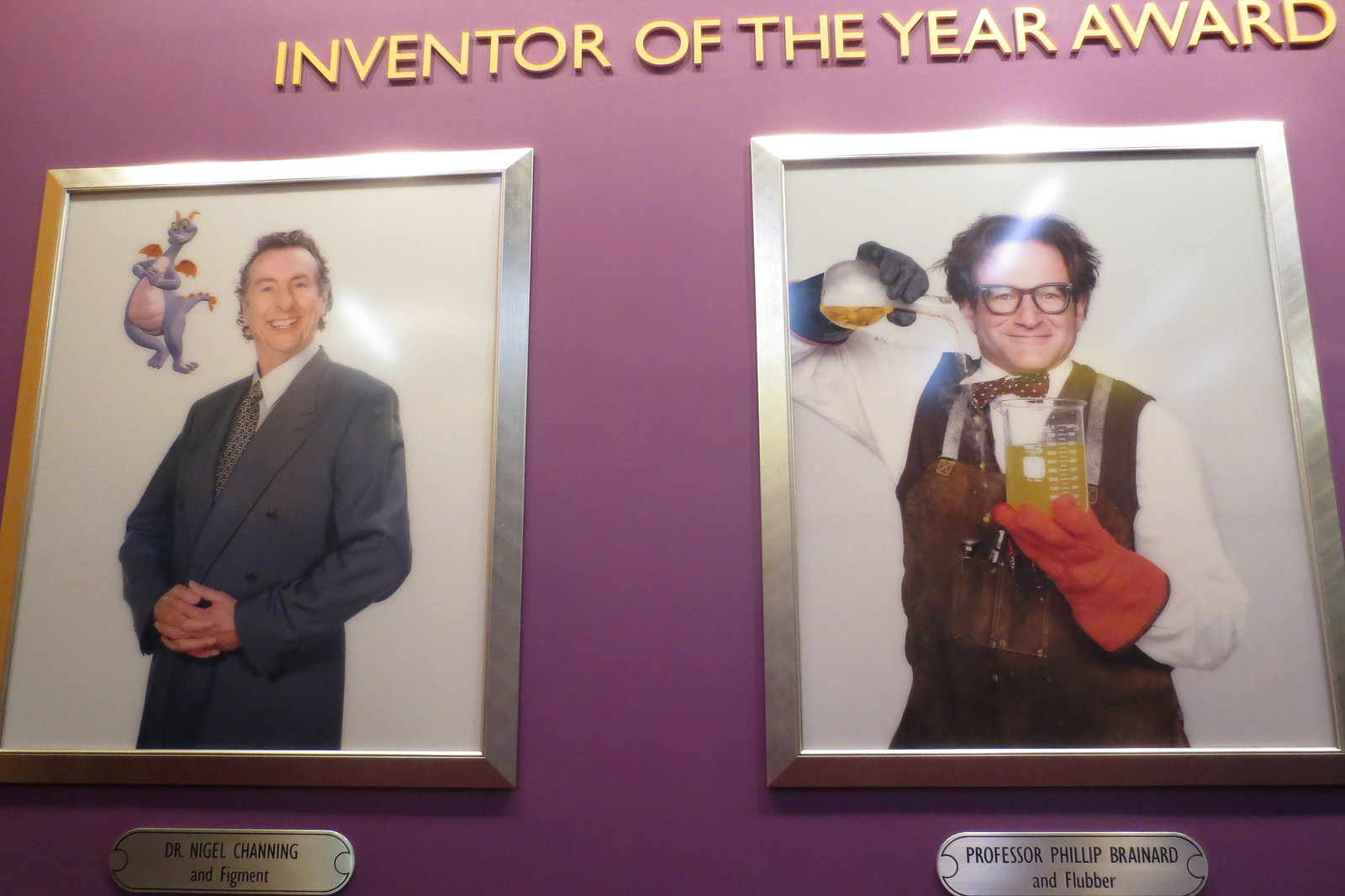The image depicts an Inventor of the Year Award display on a purplish wall. At the top, gold metallic letters spell out "Inventor of the Year Award." Below the letters are two large silver-framed photographs with name plaques. 

On the left is a formal portrait of a man with slicked-back brown hair, wearing a gray suit jacket and a darker tie, with a smile on his face. Floating beside him is a cartoon dragon, purple with a pink stomach. The plaque beneath this photo reads "Dr. Nigel Channing and Figment."

To the right is a portrait of a man resembling Robin Williams, appearing as a quirky professor. He has wild short brown hair, glasses, and is dressed in a white shirt and brown apron. He wears an orange glove and holds a beaker pouring yellow liquid, seemingly missing another beaker below. The plaque under this image identifies him as "Professor Philip Brainard and Flubber."